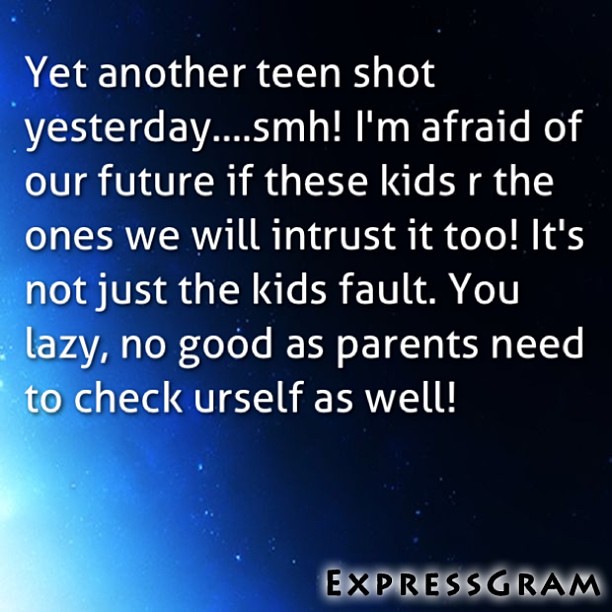The image features a gradient background that transitions from nearly black in the upper right-hand corner to a bright, almost white glow in the lower left-hand corner, resembling a starry night sky. Small white dots scattered across the background mimic stars, enhancing the celestial theme. Superimposed over this visually striking backdrop are lines of white text that convey a somber message: "Yet another teen shot yesterday... smh! I am afraid of our future if these kids, the ones we will entrust it to! It's not just the kid's fault; you lazy, no-good-as parents need to check yourself as well," with "yourself" intriguingly misspelled as "U-R-S-E-L-F." The bottom right corner features a citation in black text with a glowing white effect, reading "Expressgram."